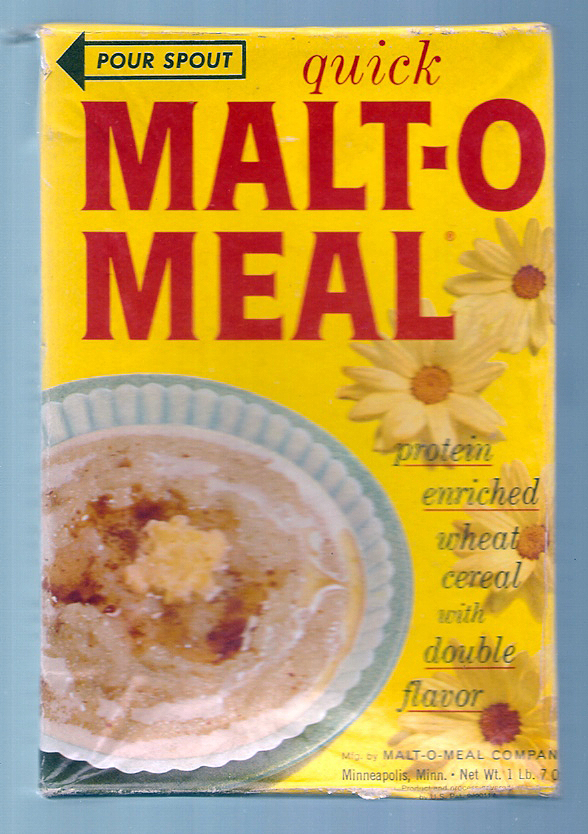The image features a yellow box of cereal labeled "Malt-O-Meal" in large, capital red letters, where "Malto" is spelled "M-A-L-T dash O" and "Meal" on the next line. The box also prominently displays the text "Quick" in red letters, signaling the product's instant preparation. In the top left-hand corner, a black arrow indicates the pour spout of the box. 

Adjacent to the Malt-O-Meal branding are two yellow flowers, adding a touch of visual appeal. Below this, in blue text with red underlines, it reads "Protein Enriched Wheat Cereal with Double Flavor." 

The lower section of the box features a white bowl with scalloped edges, resting on a blue plate, containing the wheat cereal that appears light brown in color with a pat of butter in the middle and possibly sprinkled with cinnamon sugar. Additional text in the bottom corner provides company information: "Malt-O-Meal Company, Minneapolis, Minnesota," along with "Net Weight: one pound."

The background of the image is grey, and the box's right-hand side showcases more flowers and descriptive text about the product, enhancing the box’s detailed presentation.